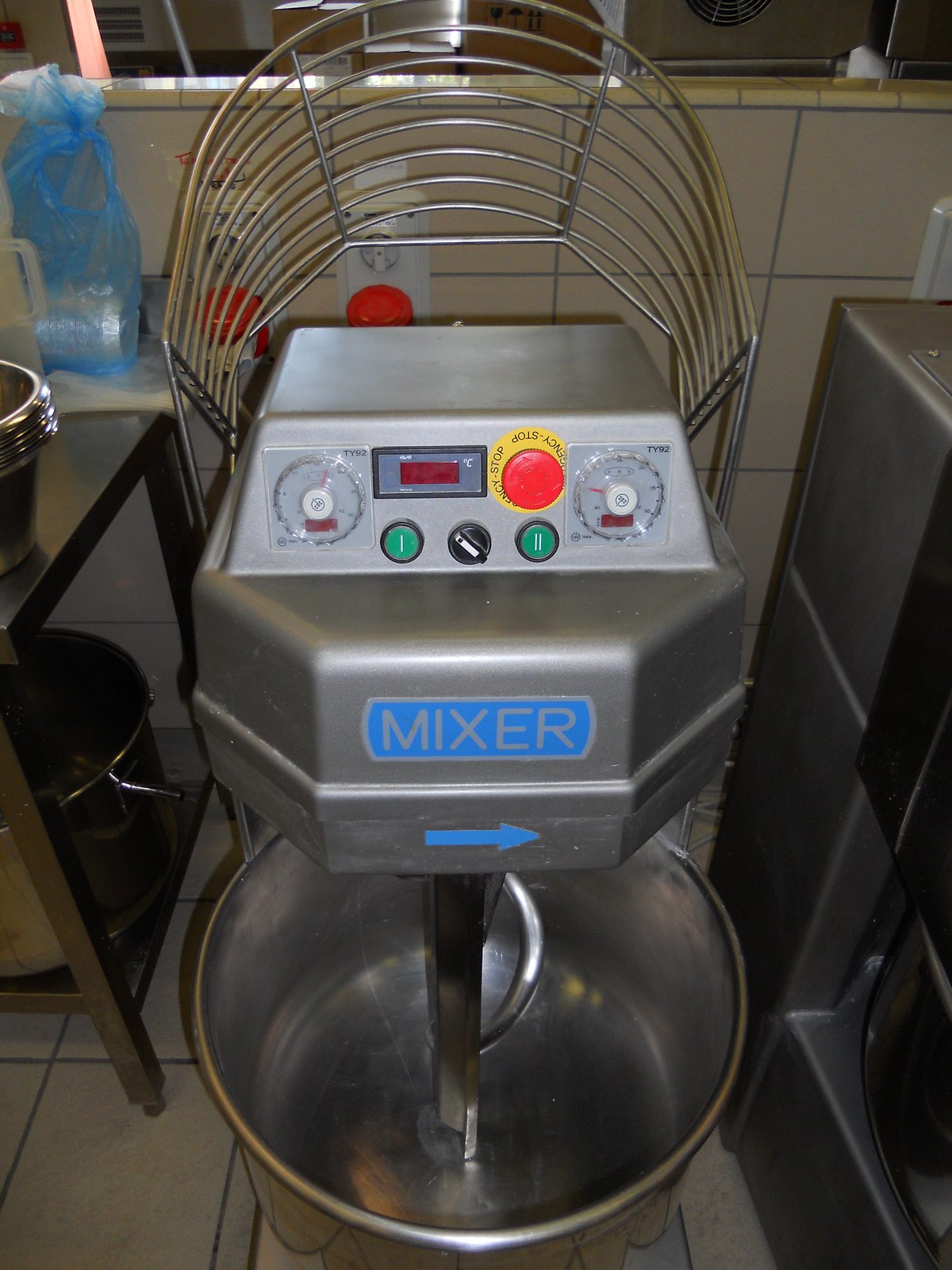This image depicts an industrial kitchen featuring a prominent silver mixer, which is labeled "mixer" in blue with a directional arrow pointing to the right. The mixer stands out against a backdrop of ceramic tile walls, characterized by white tiles with blue grouting. Above the mixer is a detailed control panel with various buttons and gauges, including green and red buttons, as well as a digital thermometer. Below the mixer, a large silver mixing bowl sits on the floor.

To the left side of the mixer is a black table or cart with visible wheels, holding a stack of silver pots and a large pot on the lower shelf. There's also a small white countertop with a tied-up light blue plastic bag. To the right side, partially visible, is another piece of furniture that includes silver shelving and additional bowls. The overall scene suggests a well-equipped, functional industrial kitchen environment.